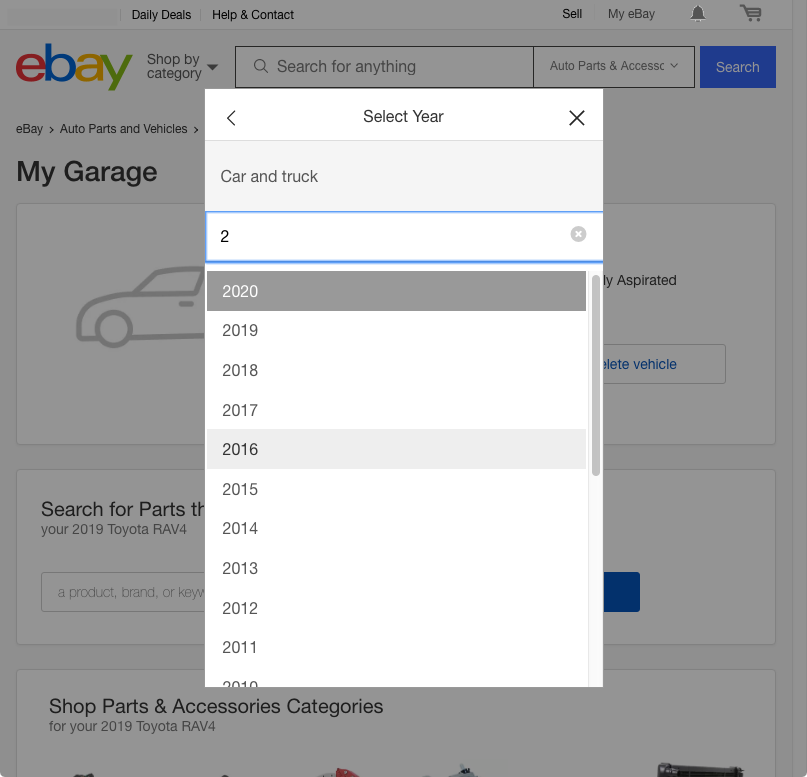This screenshot from eBay displays the homepage tailored for auto parts and accessories. On the top left, the eBay logo is prominently visible. Below the logo, the selected category is "Auto Parts and Accessories," with a blue search button adjacent to it. Dominating the screen is a large pop-up window prompting the user to "Select Year" of their vehicle in a gray bar, currently hovered over the year "2020." Behind this, the "My Garage" section showcases a sketch of a car and an option to search for parts. Partial text reading "Your 2019 Toyota RAV4" is visible, indicating that a previous search was made for this vehicle.

Underneath, there is a search box for refined searches, along with more black text on a white background stating "Shop parts and accessories" and "Categories for your 2019 Toyota RAV4." The page header features various navigational options including "Daily Deals," "Help & Contact," "Sell," "My eBay," a bell notification icon, and a shopping cart icon. The pop-up selection box includes a close (X) button at the top right corner and a navigation arrow at the top left corner.